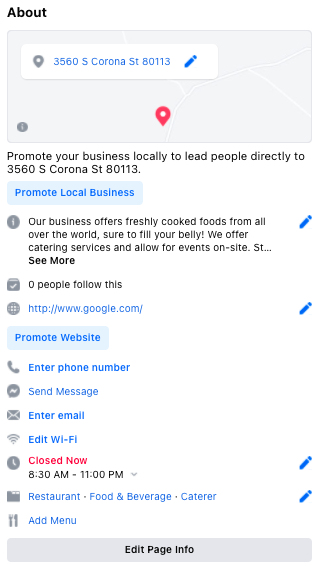**Caption:**

The image is a vertical screenshot showcasing a business listing and promotional options. At the top, bold black text reads "About." Below, a grayscale Google Maps view highlights a specific location with a red pin situated at a road that splits off. A white info box features a gray location marker and the address "3560 South Corona Street 80013" in blue text, accompanied by a blue edit icon.

Further down, promotional text advises: "Promote your business locally to lead people directly to 3560 South Corona Street 80113." This is followed by a light blue button with "Promote local business" in darker blue text.

Underneath the button, regular text describes the business: "Our business offers freshly cooked foods from all over the world sure to fill your belly. We offer catering services and allow for events on site." There is an option to "see more," marked with a blue edit icon next to it.

Following this, the URL "http://www.google.com" is displayed above a button labeled "Promote website." Further options include entering a phone number, sending a message, entering an email, and editing Wi-Fi information. Below these, the business status is listed as "Closed now," with operating hours from 8:30 AM to 11:00 PM.

Lastly, categorization tags such as "Restaurant," "Food and Beverage," "Cater," and an "Add menu" option are present. The screen ends with a gray "Edit page info" button at the bottom.